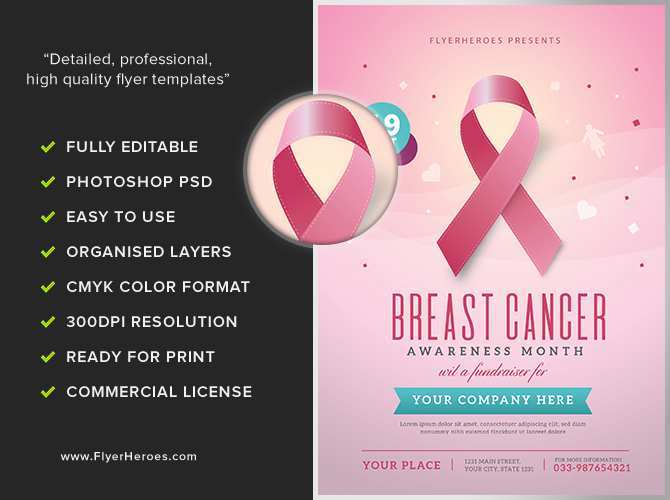The image showcases the home page of flyerheroes.com, a website specializing in providing detailed, professional, high-quality flyer templates for various occasions. 

On the left-hand side of the image, there is a gray rectangle containing a series of bullet points that emphasize the key features of the templates offered by Flyer Heroes: 
- Fully editable
- Photoshop PSD format
- Easy to use
- Organized layers
- CMYK color format
- 300 dpi resolution
- Ready for print
- Commercial license

Additionally, the gray rectangle includes the company’s slogan, "Detailed, professional, high-quality flyer templates," and the website URL: www.flyerheroes.com.

On the right-hand side, there is a slightly larger rectangle showing an example of one of the available flyer templates. The pink flyer is designed for Breast Cancer Awareness Month and features a crest in the center. Below the crest, the flyer states "Breast Cancer Awareness Month" and "Fundraiser for [Your Company Name]," demonstrating how businesses can customize the template to suit their specific needs. The example highlights the professional and polished look that can be achieved effortlessly using Flyer Heroes' templates.